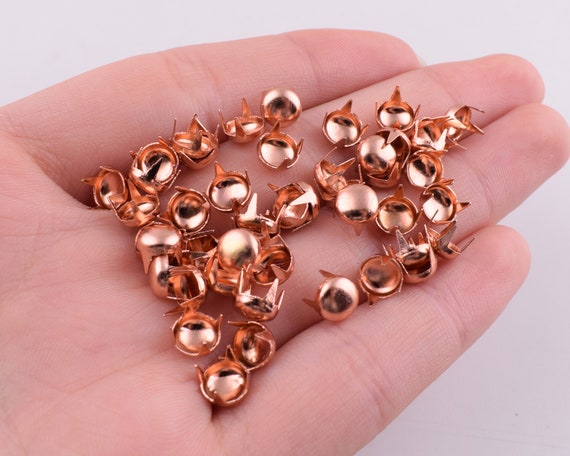This is a detailed photograph of a Caucasian person's hand, which has a pale pinkish hue showcasing visible veins and a unique handprint. Nestled in the hand are approximately 20 to 30 small pins, each with a rose gold dome top and four sharp legs that can puncture or attach to crafting projects. The pins, described as having a light orange-ish pink color, appear as numerous small dots scattered across the palm.